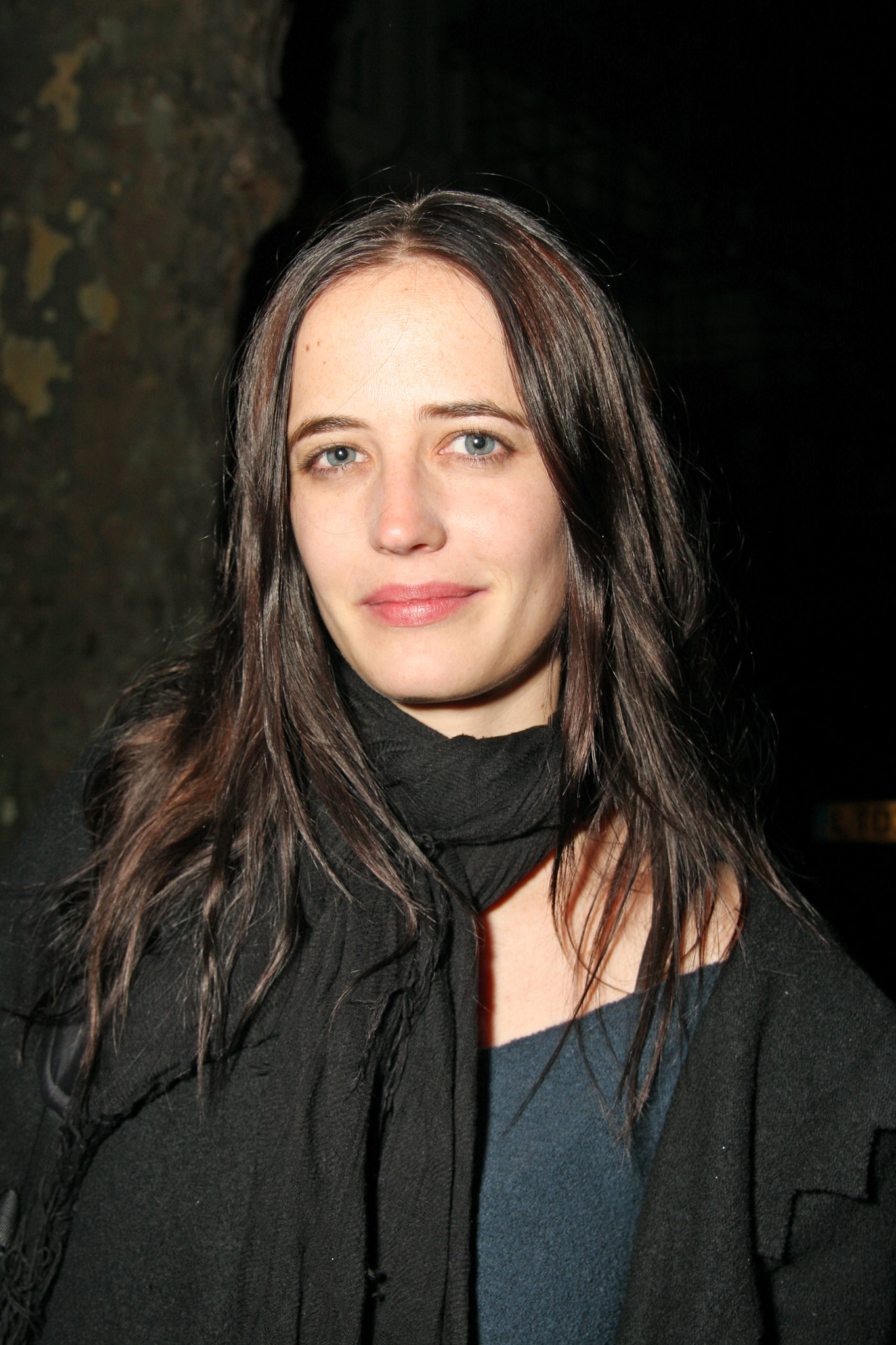This photograph captures a younger woman with straight, long dark brown hair that cascades below her shoulders and features subtle reddish-brown highlights. Her captivating blue eyes, tinged with greenish hues, stand out against her smooth complexion. She wears a delicate application of light red, almost pink, lipstick, and her expression is serene with a closed-mouth smile. The woman is dressed in a dark blue sleeveless top, layered with a black felt coat, and wrapped around her neck is a thin, soft black scarf. Her attire creates a harmonious dark ensemble, which complements the mysterious black background. To the left side of the image, part of a natural stone rock with light brown spots is visible, adding an earthy element to the otherwise dark and focused composition. This detailed portrayal gives a sense of both the woman's graceful appearance and the subtle, natural detail of her surroundings.